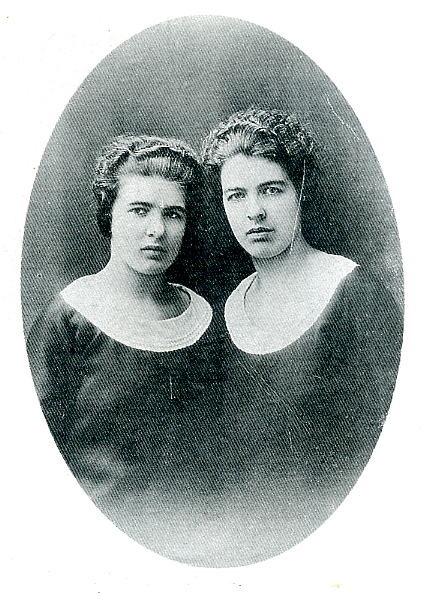In the center of this oval-framed, antique black and white photograph, set against a solid white background, are two dark-skinned young women in their late teens or early twenties, likely sisters judging by their strikingly similar facial features. Captured possibly in the late 19th or early 20th century, the women are positioned with the shorter woman on the left and the taller woman on the right. Both have tightly kinky hair styled back in a wavy pattern and wear identical black dresses resembling robes with wide sleeves and large, white-trimmed low necklines. Their expressions are serious and somber, almost troubled, with no trace of a smile. The image itself shows signs of age with slight scratches or cracks marring its surface, enhancing the sense of historical depth.